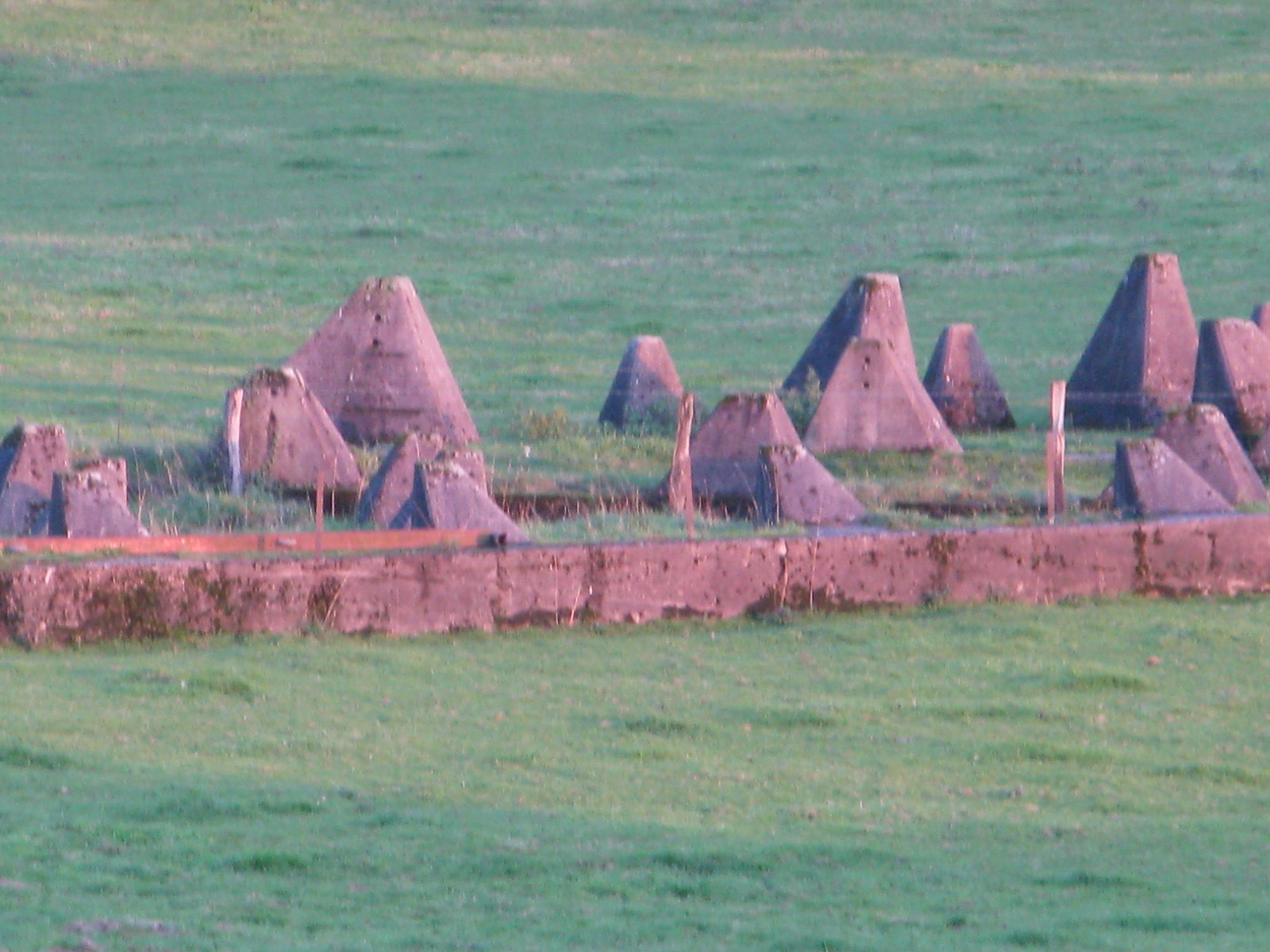This photograph depicts a series of strange, pyramid-shaped stone structures stretching horizontally across the entire middle third of the image, against a backdrop of a short, somewhat uneven grassy field. The stones, which appear almost pinkish due to the light—suggesting the photo was taken either in the morning or late afternoon—are of varied sizes and shapes, with some taller, oblong, and broken at the tips, while others are smaller but equally irregular. There are about a dozen of these structures, haphazardly scattered, without any specific order. A low stone platform, slightly overgrown with moss, supports these formations, and in front of it, is a fence made of wooden posts and wire, offering some scale to the scene. The image quality is notably low, with visible color distortions and a sense of weathering, as if the photograph had been copied or stretched multiple times.